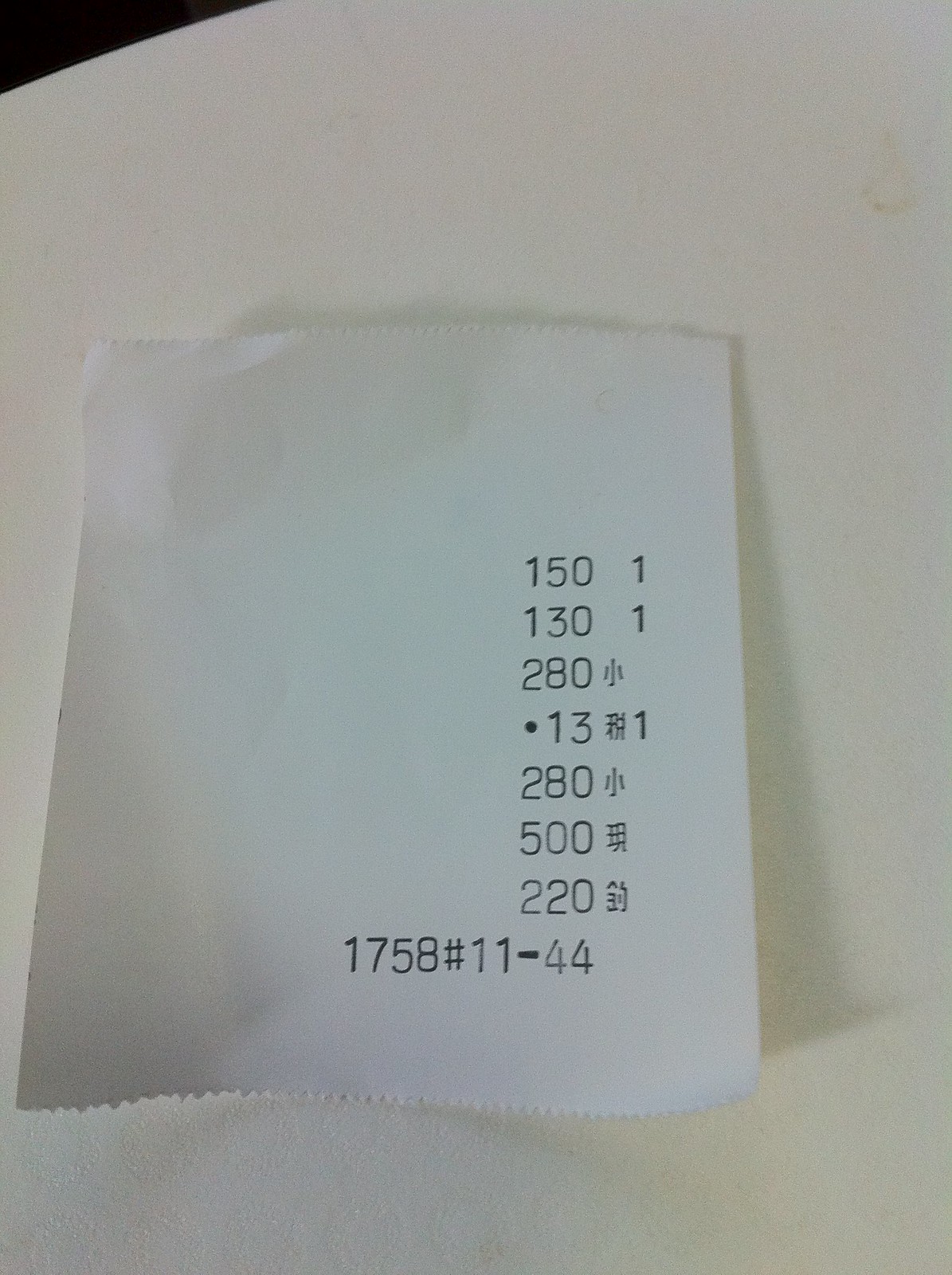The photograph captures a high-resolution image of a receipt prominently featuring Japanese characters, making the specific currency and denomination indiscernible to non-Japanese readers. The receipt, made from traditional receipt paper typically used in printer rolls, measures approximately three inches in width with serrated edges at both the top and bottom, suggesting it was manually torn from a cash register or printer. The white paper receipt lies curled slightly against a pristine white background, casting a faint shadow beneath its gently bent form.

The receipt displays a vertical list of numbers: 150, 130, 280, 13, 280, 500, and 220, each accompanied by various Japanese characters, likely indicating item descriptions or categories. At the bottom of the receipt, the total sum appears to be 1758, followed by a pound sign and the time 11:44. The detailed alignment and legibility of the print suggest the receipt was recently produced, preserving its crisp texture and clean edges against the minimalist setting.